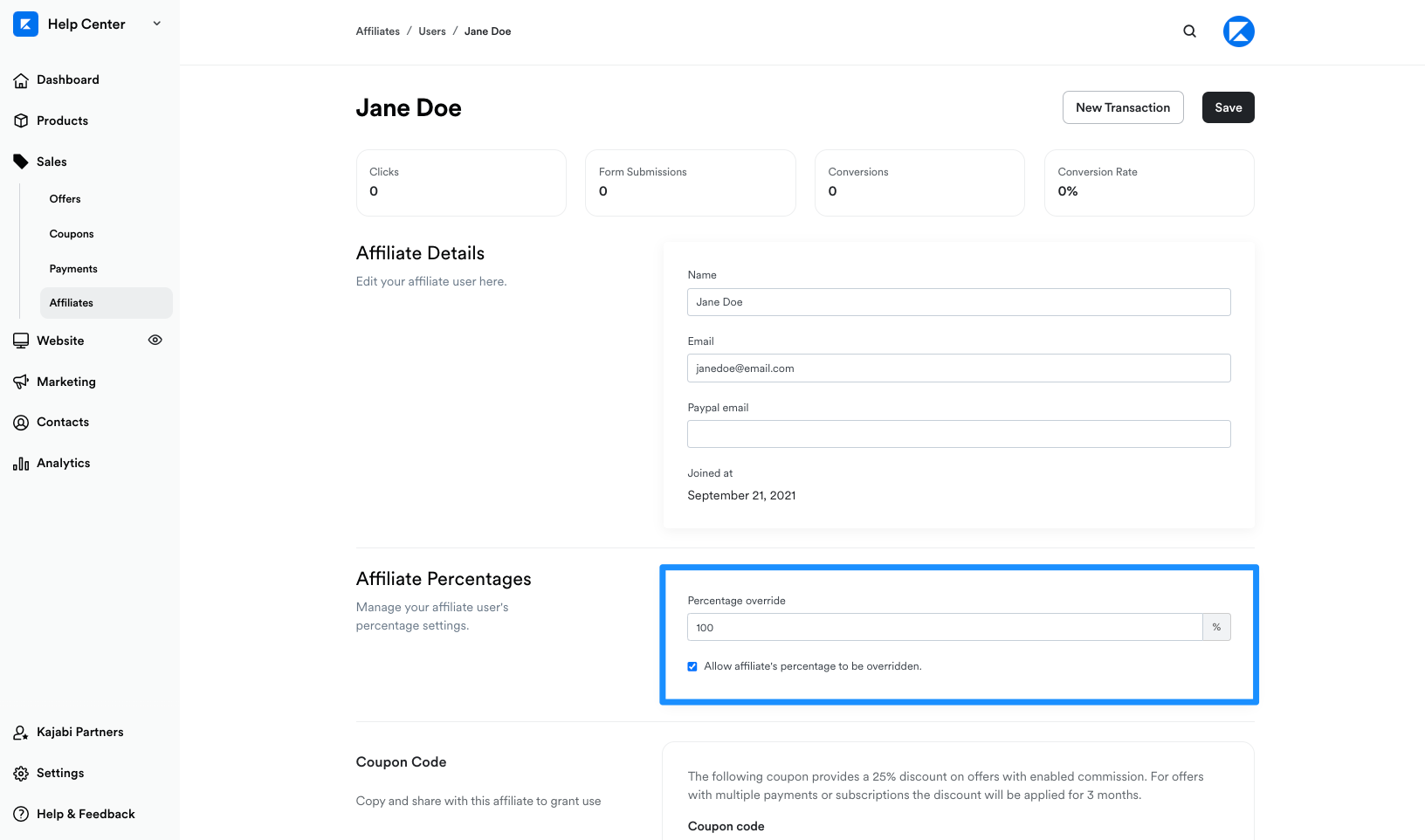Screenshot Description: The image captures a Help Center page from an unspecified app or website. On the left-hand side, a gray vertical menu bar displays several key sections, listed as Dashboards, Products, Sales, Website, Marketing, Contacts, and Analytics. 

The main content area showcases an example page titled "Jane Doe," which organizes information under subheadings such as Affiliate Details, Affiliate Percentages, and Coupon Code. Each of these subcategories includes editable fields where users can input data like Name, Email, PayPal Email, and Percentage Override, along with an option to enter a Coupon Code. Additionally, a prominent button labeled "New Transaction" is visible on the page.

Despite the detailed layout and multiple sections, the specific platform being used remains unidentified.